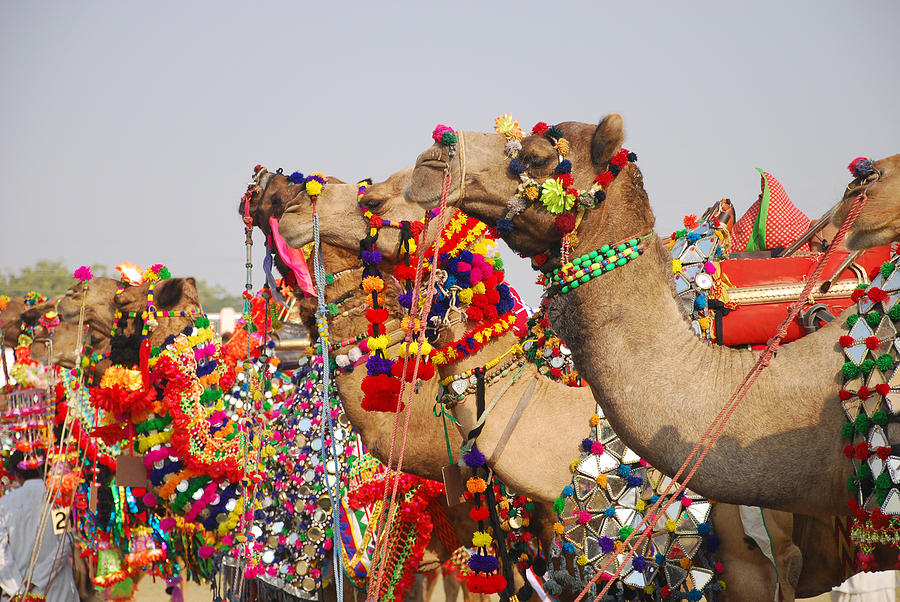This captivating photograph features a group of five camels adorned with an array of vibrant decorations, creating a highly colorful and festive scene. The camels are standing in close proximity to one another, with their heads held high, giving them a regal appearance. Each camel is draped in intricate ornaments, including necklaces, garlands with pom-poms, and elaborate headdresses. The adornments feature a spectrum of colors—reds, greens, yellows, whites, pinks, oranges, purples, and even rainbow hues. 

The nearest camel to the camera has its eyes shut and is covered in various beaded necklaces and small decorative mirrors. All camels are decorated elaborately around their necks, faces, and backs, with their vibrant trappings including red harnesses and reins, suggesting they are posed for the photo. The reins, also decorated with bright pom-poms, lie in front of the camels, who stand stoically with their mouths closed.

In the background, a hazy, smoky sky is visible with some green trees, adding a serene contrast to the colorful spectacle in the foreground. On the far left, a person clad in what appears to be a white robe can be seen, adding a further dimension to the festive, almost ceremonial atmosphere of the image.